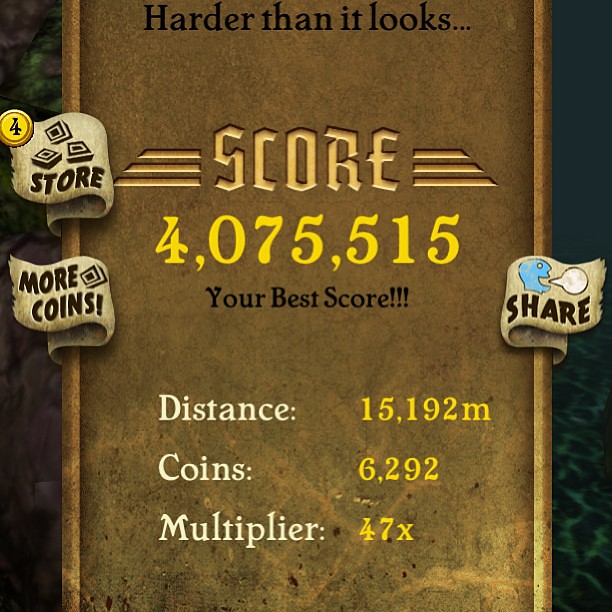The image is a screenshot from a mobile game, displaying a detailed score screen with a bluish and greenish border on the left and right sides. At the top, it reads "Harder than it looks..." in black text. The centerpiece is a gold rectangular object that highlights the player's achievements in different colors: the main score "4,075,515" in yellow, labeled "Your Best Score" in gold, the distance of "15,192 meters" in white, the number of "Coins: 6,292" in white, and a multiplier of "47x" in white. Alongside the score screen, on the left, there is a white icon featuring three squares with a small number "4" above it and the text "Store" and "More Coins" below. On the right side, there's an image of a blue head with a text bubble indicating "Share." The overall background behind the score screen appears to be a teal color.